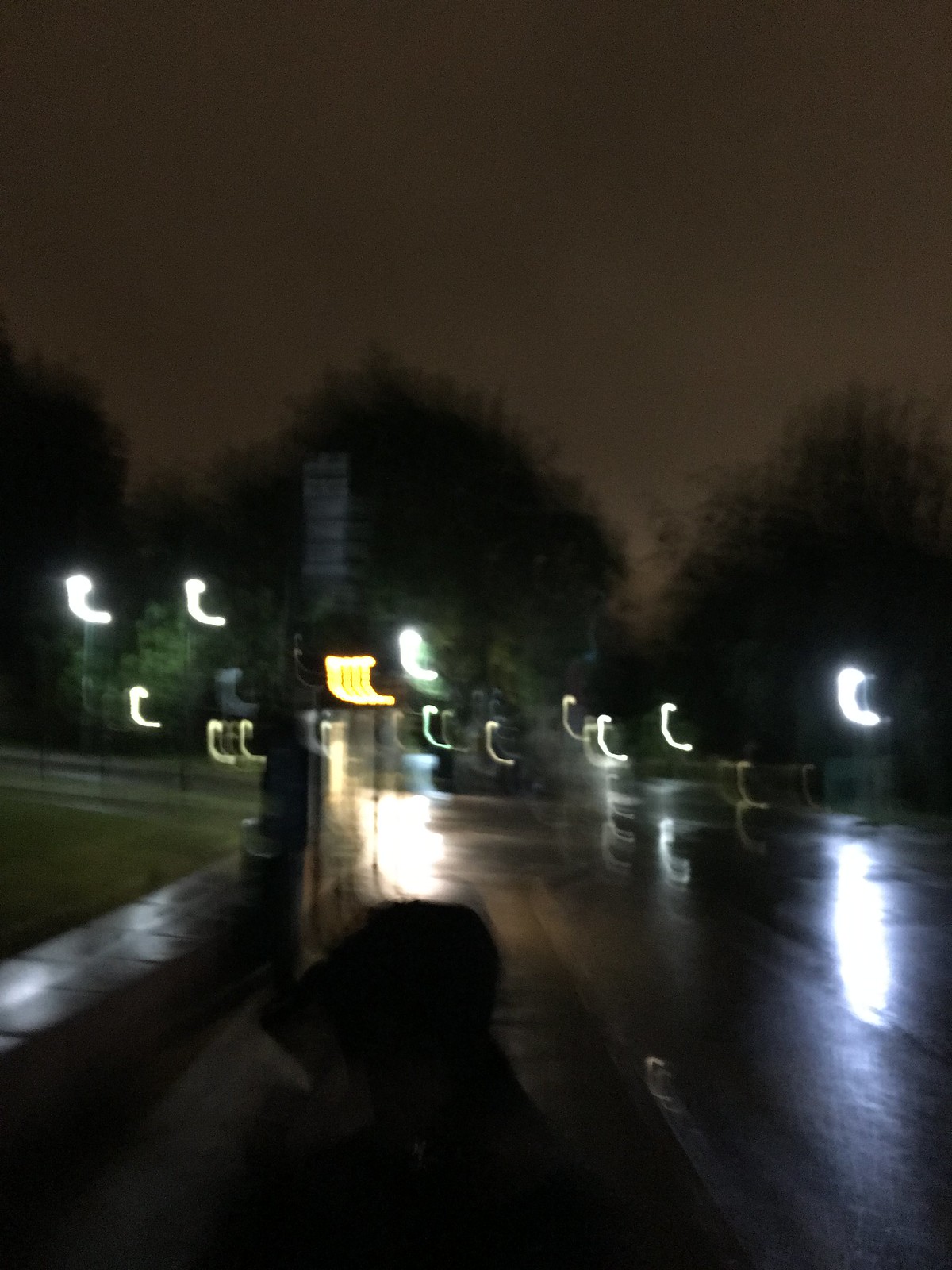In this double-exposed photograph, a nighttime intersection is depicted, imbued with a dreamlike quality due to its blurriness. The wet streets reflect the ambient light, creating a shimmering pathway that leads into the distance. Dominating the scene is a lit-up kiosk or street sign, though its message remains unreadable due to the blur. The glowing golden lights on the kiosk are striking, arranged in horizontal, C-shaped patterns. 

In the foreground, there is a dark, indistinct figure that appears almost mechanical, adding an enigmatic element to the image. The main street extends straight ahead with a secondary street branching off to the left, both dotted with streetlights that emit the same C-shaped light streaks due to the double exposure.

To the left of the illuminated kiosk, a wet sidewalk with distinctive-looking bricks can be seen, flanked further left by a grassy boulevard. In the far background, several trees stand tall, their green, leafy canopies visible even in the night. The entire scene is bathed in an ethereal glow, captured eloquently by the interplay of light, shadow, and the reflective wet surfaces.